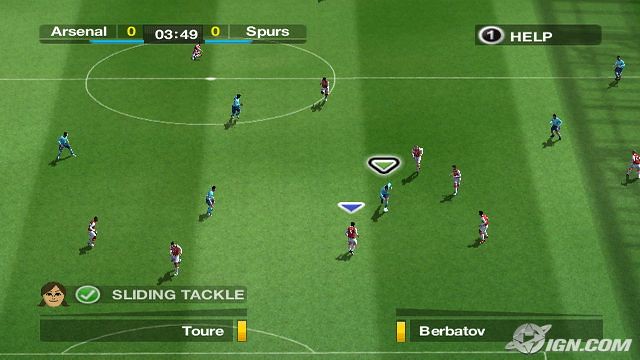This image captures a scene from a soccer video game featuring a match between two teams - Arsenal and Spurs. The players are dispersed across a lush green field, with the two opposing teams identifiable by their red and blue uniforms. 

In the upper left corner, a scoreboard reads "Arsenal 0" and shows that 3 minutes and 49 seconds have elapsed, with "Spurs" also at 0. This indicates that the game is currently tied. 

On the bottom left, there's a small icon of a cartoon woman's face next to a green checkmark, accompanied by the text "Sliding Tackle" and the name "Toure" highlighted on a green bar beneath it. There is a small yellow rectangle next to this segment.

On the right side of the screen, a black bar features the number "1" enclosed in a circle, followed by the word "Help."

In the lower right corner, another yellow rectangle appears above a green bar displaying the name "Berbatov." In the extreme lower right corner, a logo resembling a planet with a ring around it, possibly Saturn, is visible along with the text "IGN.com," indicating branding or a watermark from the website.

Overall, the vibrant colors and detailed HUD elements aptly convey an immersive and interactive soccer gaming experience.